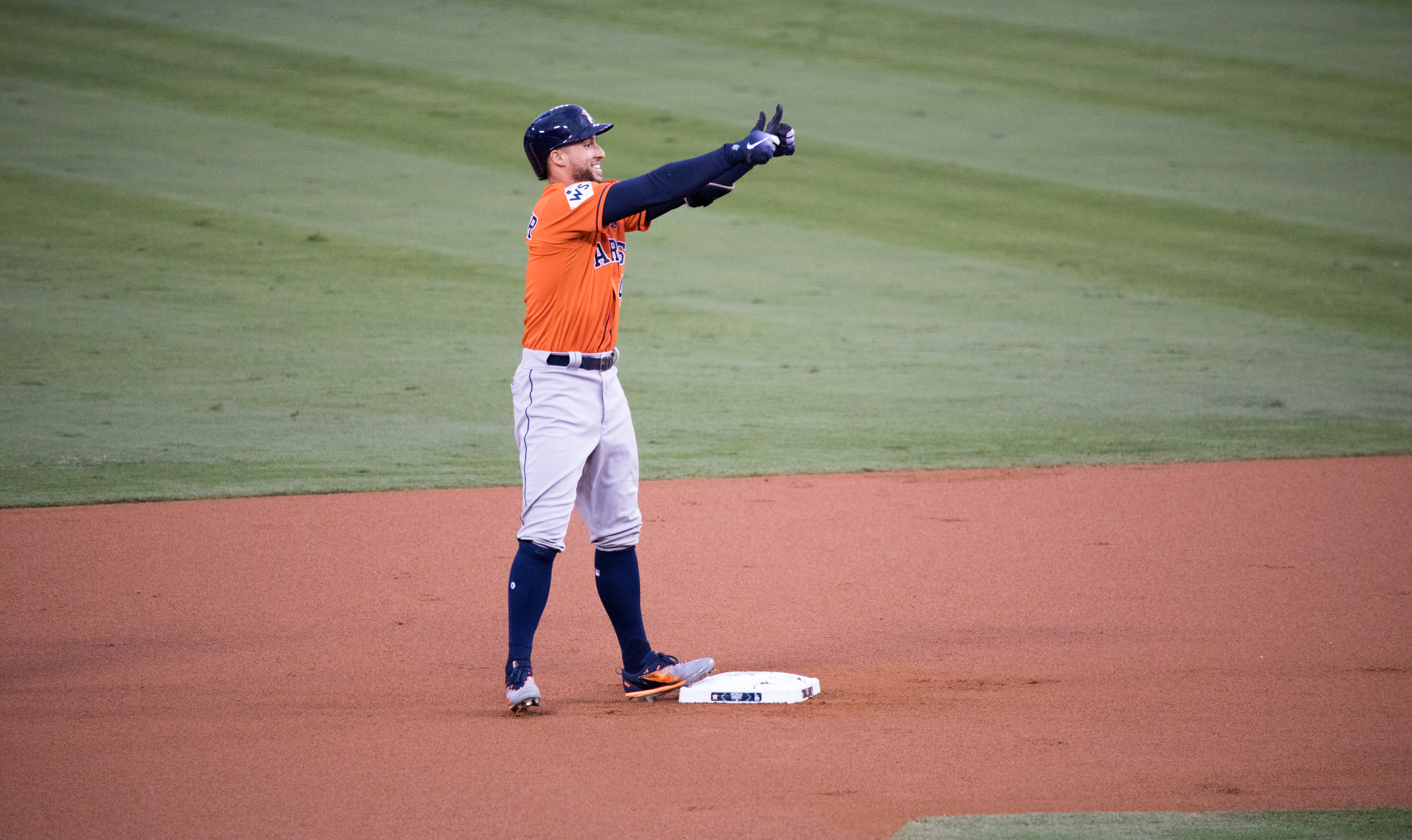This detailed photograph captures a smiling baseball player standing prominently at the center of a baseball field. He is dressed in a vibrant orange, white, and blue uniform with blue lettering on both the front and back of his jersey. A white logo adorns his navy blue hard-shell baseball cap, and a marking that appears to be "W5" or "WS" is visible on his right shoulder. The player is positioned adjacent to a white base, specifically third base, with his left foot placed on it while his right foot remains off the base. His arms are raised high, giving two enthusiastic thumbs up as he smiles, likely at someone off-camera. The background reveals the distinct red dirt of the baseball diamond and a large expanse of freshly mowed grass, highlighted by visible mowing lanes, indicating an outdoor setting in the middle of the day. The colors prominently featured in this image are blue, orange, white, brown, and green.